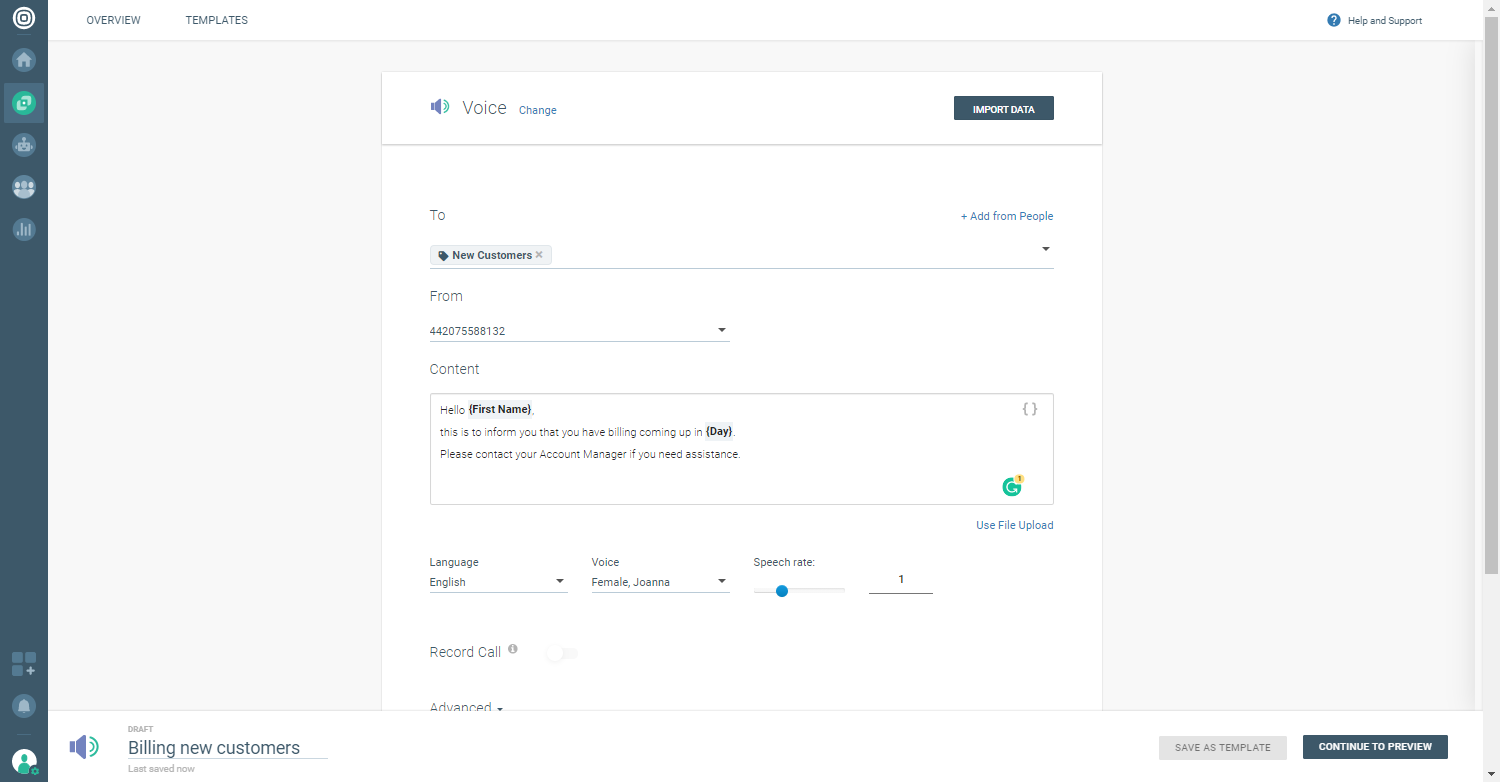The image depicts a detailed sign-up page with a form situated prominently in the center. The site menu is located on the left side, featuring dark blue tabs. At the top, there are additional tabs labeled "Overview" and "Templates." Towards the top-right corner, there are options for "Help" and "Support." 

In the bottom left corner, there's a status indicating "Draft, building new customers, last saved now," alongside an image of a blue and green speaker. At the top-center of the form, "Voice Change" is displayed, with an "Import Data" button in dark blue to its immediate right. The form's background is predominantly white.

Within the form, there's a section labeled "To" with a link titled "Add from people" on the right side. Below it is a field labeled "From" with the number "442075588132" entered. Further down, a "Content" section reads: "Hello, [First Name], this is to inform you that you have billing coming up in the day. Please contact your account manager if you need assistance." A green Grammarly icon for "Search" is positioned at the bottom-right of the text field, and there's an option for "Use file upload."

At the bottom of the form, language settings are displayed as "English," with the voice set to "Female Joanna" and a speech rate of "1." Options like "Record call" and "Advanced" are also noted, indicating that this is a record call page. Finally, in the bottom-right corner, there are two buttons: "Save as Template" in grey, and "Continue to Preview" in dark blue.